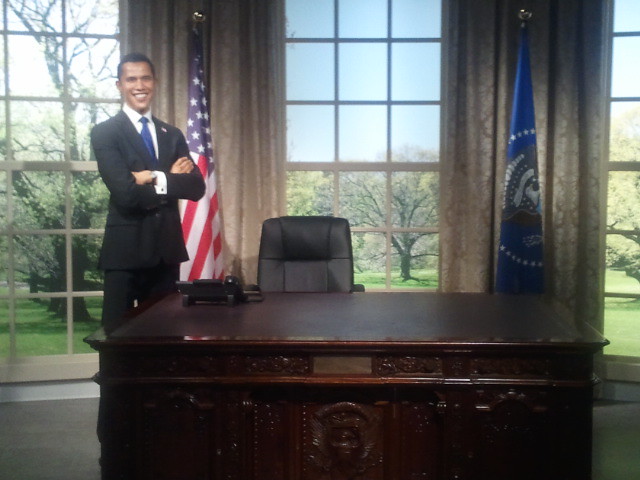The photograph depicts President Obama in the Oval Office. He stands beside a majestic, dark, shiny mahogany desk adorned with intricate wooden carvings at the front. On the desk, there is only a black phone. President Obama, a thin man with darker skin and short black hair, is dressed in a black suit, white collared shirt, and blue tie. Behind him are the U.S. flag and another blue flag featuring an eagle. The office space is framed by beige curtains and large windows that provide a view of lush trees and grass outside. A black chair is placed behind the desk, adding to the formal atmosphere of the room. The detailed elements, combined with the decor and flags, clearly indicate that this scene is set in the Oval Office.